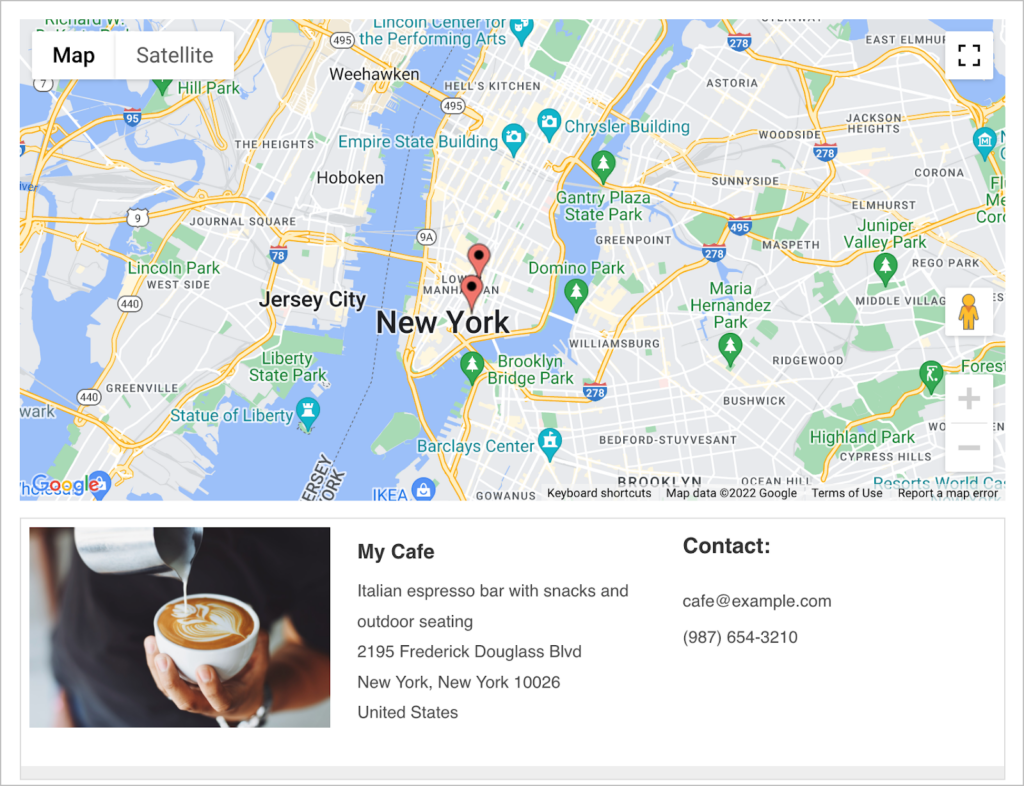Here’s a cleaned-up and detailed caption for the image you described:

---

The image showcases a web-based map interface, prominently featuring New York City. In the upper left corner, there's a black, bold "Map" label next to a thin separator line, followed by a light gray "Satellite" option. The main portion of the map is centered on New York, illustrating the city's layout with visible bridges extending into New Jersey, including Jersey City at the top edge.

This map appears to be computer-generated, similar to what one might find on Google Maps. Two marked points of interest highlighted with red GPS signals are visible around Lower Manhattan. Below these markers, there is a featured image depicting a person's hands pouring cream into a cup of espresso, creating a delicate design in the foam. Accompanying this visual is a text box labeled "My Cafe: Italian Espresso Bar with Snacks and Outdoor Seating" and the establishment's address and contact information.

---

Thank you for watching!